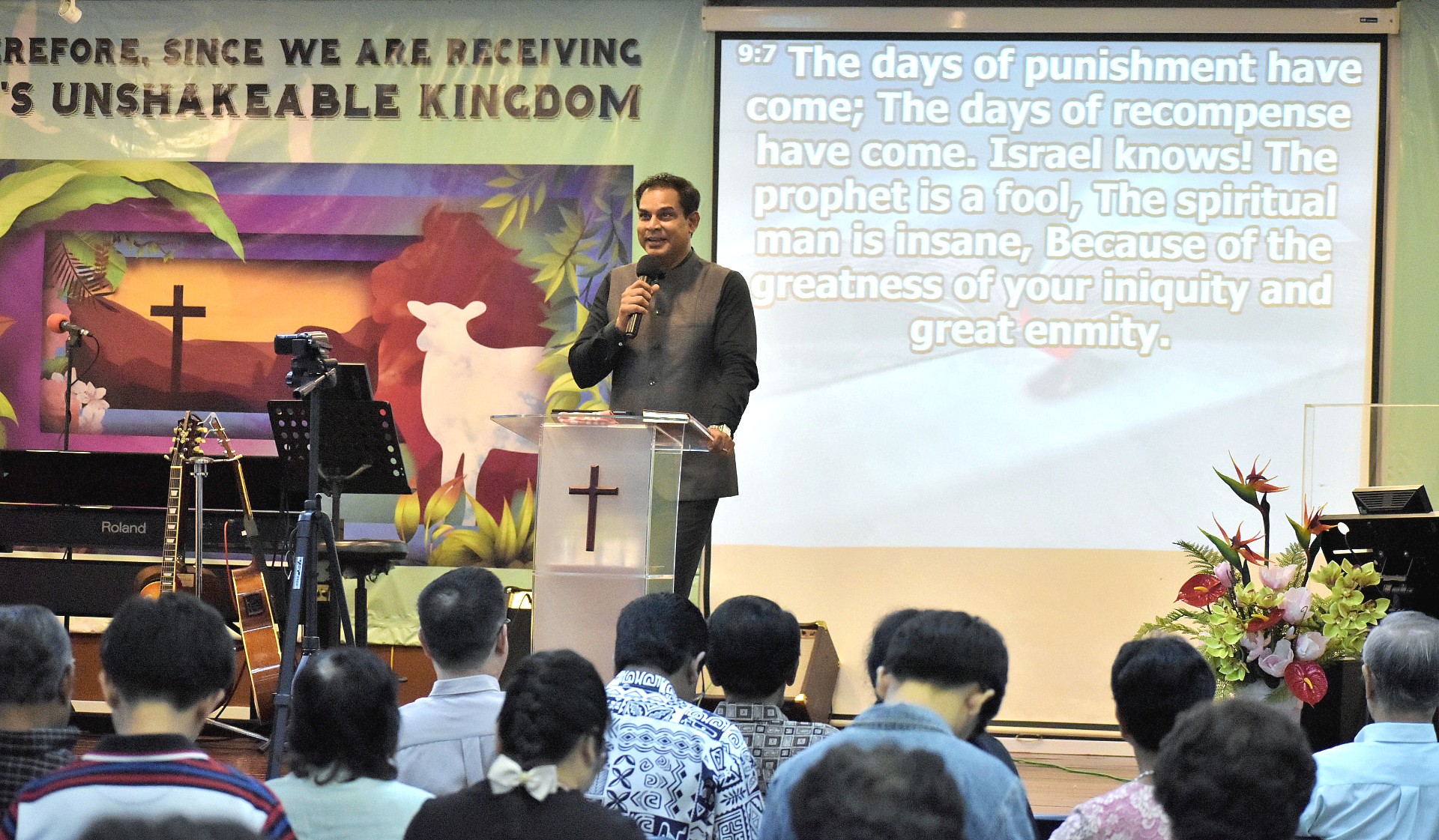The photograph captures a detailed moment of a man, possibly a pastor, giving a presentation or sermon in a church setting. Centered in the landscape view, the man, who appears to be of Middle Eastern or Indian descent with a tan complexion and short light brown hair, is dressed in a black shirt, gray vest, and black pants. He is holding a black microphone in his right hand and has his left hand resting on a clear, glass lectern, which features a dark brown wooden cross at the front.

Behind him, a projection screen displays a passage in white text against a blue background: "The days of punishment have come, the days of recompense have come. Israel knows the prophet is a fool. The spiritual man is insane because of the greatness of your iniquity and great enmity." The screen is mounted on a green wall, and to its upper left side, a poster partially visible reads, "since we are receiving unshakable kingdom". The poster is adorned with vibrant imagery, including a white animal, likely a lamb, looking towards a black cross set in a desert landscape with dark red hills, orange wash, and green leaves, all accentuated with blue and purple lines.

In the foreground, the heads of the audience members are visible, indicating a group attentively listening to the speaker. To the right of the poster and slightly above the heads, musical instruments such as a piano and a guitar are present but unplayed. The overall ambiance is well-lit, providing clarity and highlighting the serene yet engaging atmosphere of the scene.